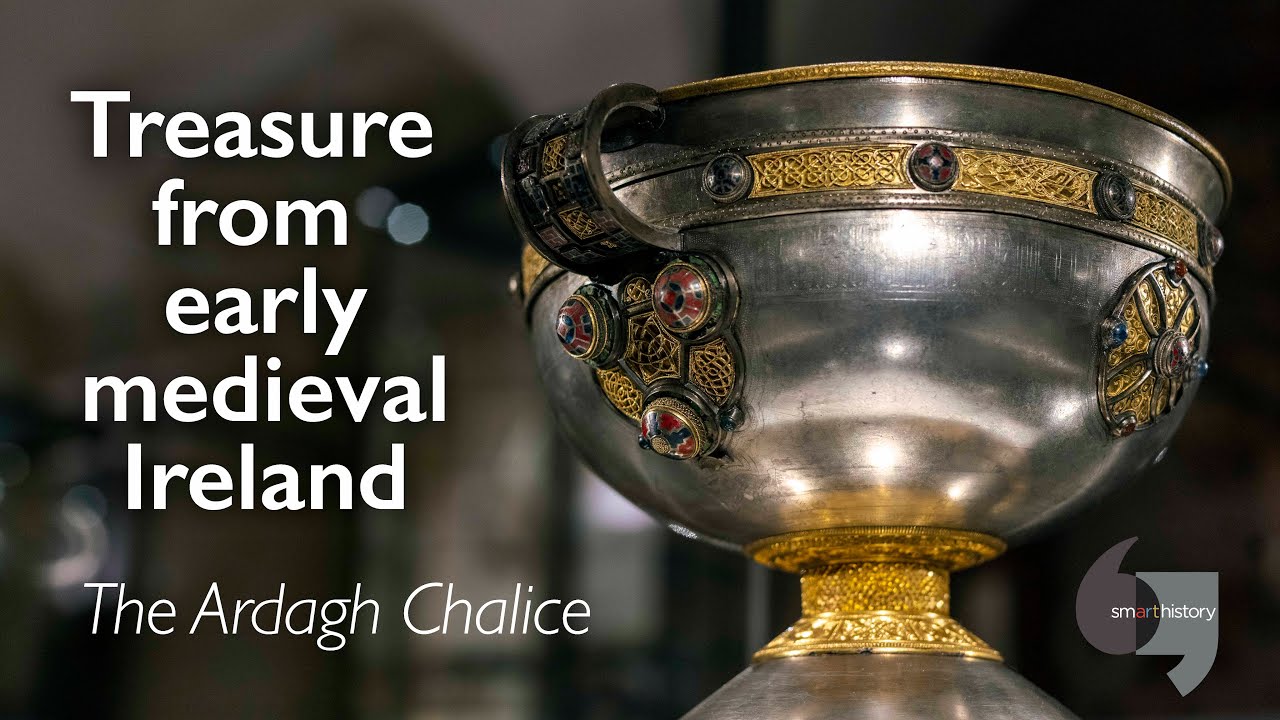This image features the Ardagh Chalice, a treasured artifact from early medieval Ireland. The chalice, predominantly silver, is adorned with numerous intricate gold details and embedded with various gemstones. It has a distinctive structure with finger holes on its side, each surrounded by elaborate carvings. The chalice is composed of multiple bands: a golden band at the top rim, another in the middle section separating the upper and lower parts of the chalice, and a third golden ring around the base. The handle is short, curved outwards, and black in color.

Decorations on the chalice include intricate gold shields and circular motifs adorned with jewels. The central circle features three red gems and smaller blue gems on either side, while a gold ring around the top edge alternates between blue and red gems. The overall design combines silver craftsmanship with detailed gold accents and the colorful sparkle of red and blue stones, creating a captivating and richly ornamented piece.

In the bottom right-hand corner of the image, a logo featuring quotation marks in shades of grey can be seen, with the text "Smart History" written above and a red 'A'. The left side of the image has text reading "Treasure from early medieval Ireland, the Ardagh Chalice." The background is blurred to keep the focus on the detailed craftsmanship of the chalice.